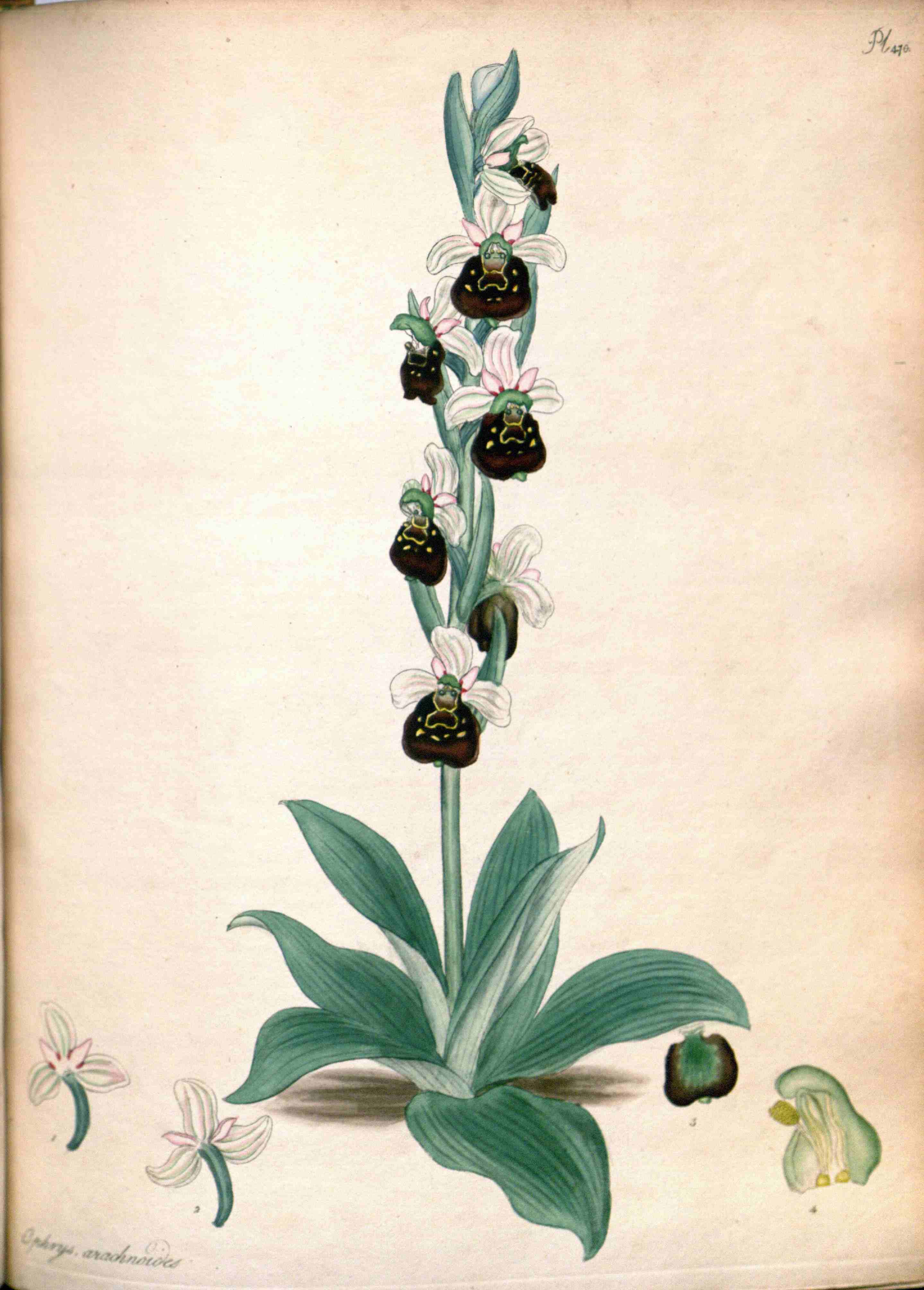This is a detailed botanical illustration of an orchid rendered on an off-white, aged paper that has a vintage feel. At the base of the plant, there is a low-growing central rosette with several large, thick green leaves that have pointed tips. A single, tall flower stalk emerges from the center, adorned with multiple blooms all the way up. Each flower features three white petals with subtle gray veining and hints of pink, along with a distinctive central dark brown, bulbous petal that has yellow specks. To the left of the main illustration, there are two close-up images showing the flower petals without the central brown petal. On the right side, the drawing includes detailed diagrams of a leaf and the intricate structure of the dark brown petal. The background is a cream or ivory color with some brownish aging, and in the top right corner, there is some small, cursive writing, likely the scientific name of the plant, penciled in. The muted green foliage and overall faded colors enhance the vintage aesthetic, consistent with traditional field identification guides.